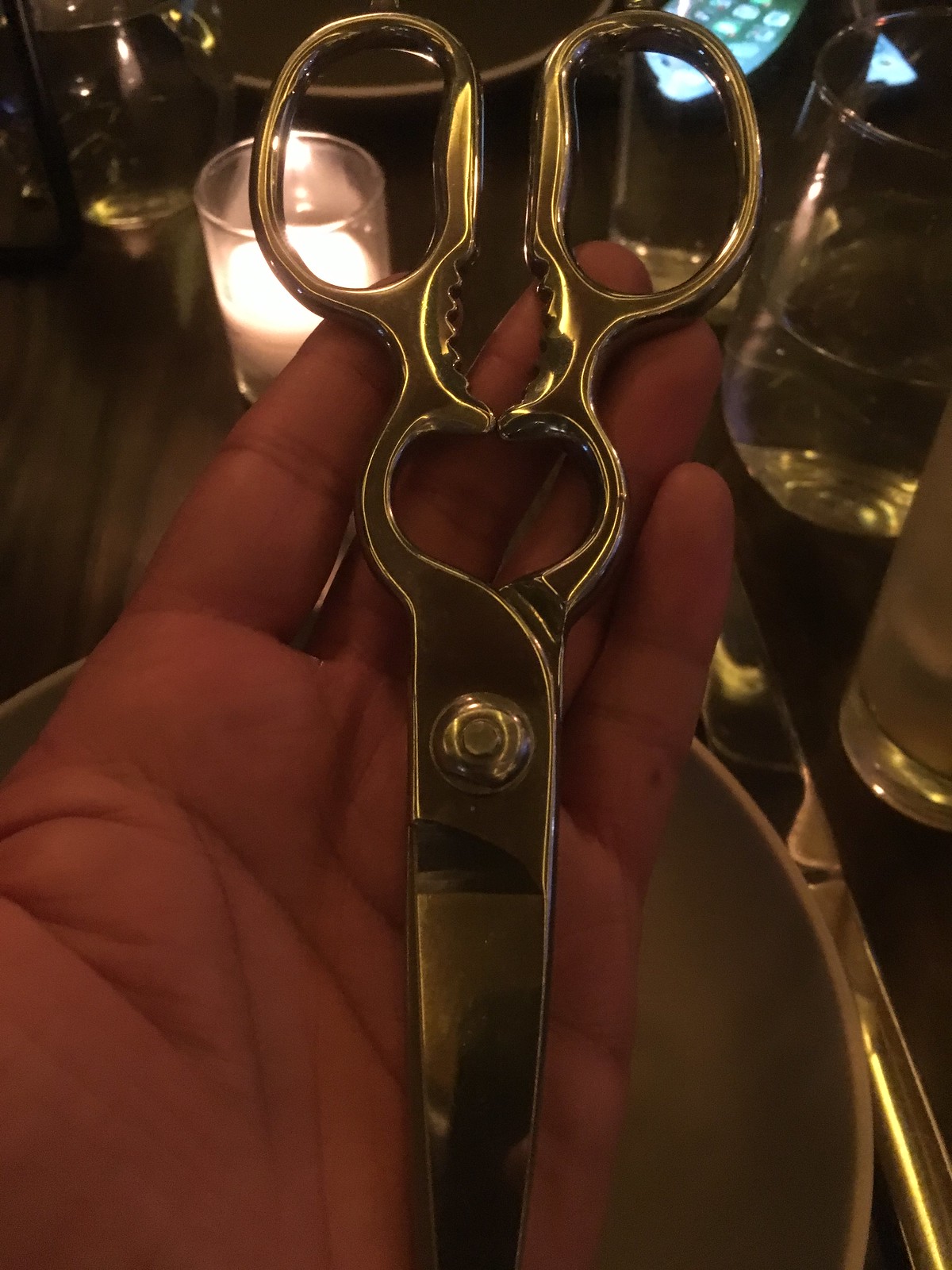In this vertically oriented, color photograph taken from above, a light-complected hand holds a pair of shiny gold scissors, lying flat with the blades pointing downward. The scissors, which might be kitchen or sewing shears, feature a serrated middle section that could function as a bottle opener, and are held together by a prominent metal rivet. The finger holes are large and flattened at the bottom, adding to their intricate design. The photograph is candle-lit, creating a warm, low-light ambiance. In the background, beneath the hand, is a white or light gray plate. To the right, there is a silver butter knife and two drinking glasses with clear liquid; one glass is full and the other is one-third full. A lit votive candle in a simple jar is positioned towards the top left, casting a gentle light over the scene. Additionally, another glass, possibly containing milk, is slightly visible behind these objects. The main focal point remains the hand and the golden scissors, with the background adding context and depth to the image.